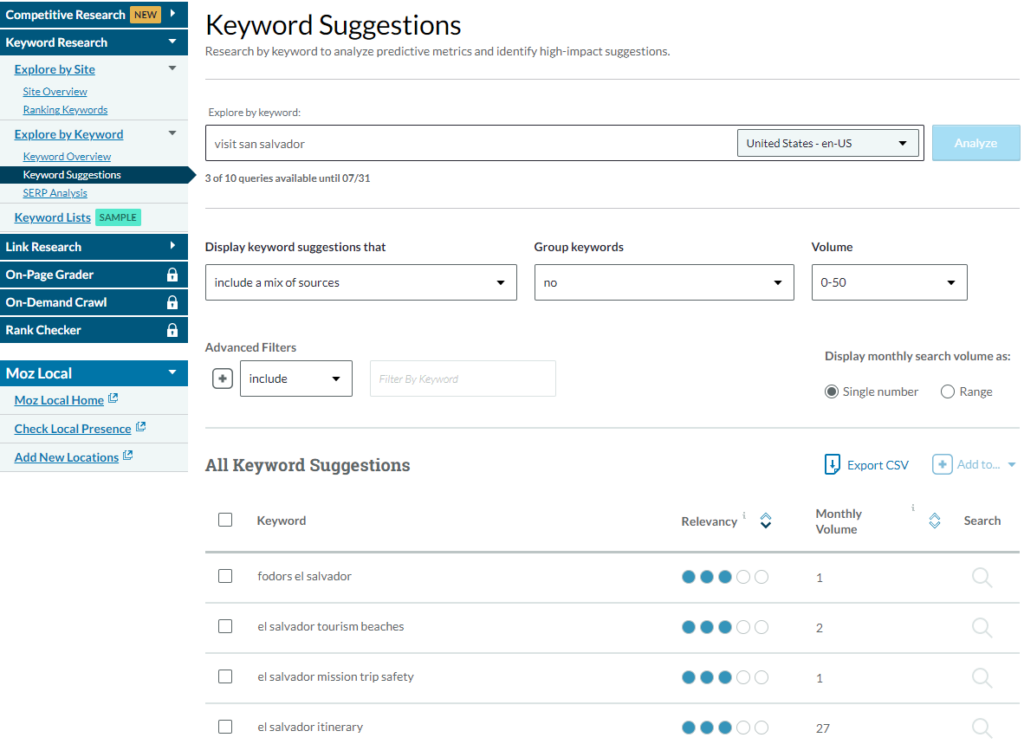The image displays a comprehensive view of a SEO software interface. 

In the top left corner, the heading "Competitive Research" is prominently displayed. Directly below it is another section labeled "Keyword Research," containing several tabs for additional options. Further, four distinct features are listed in succession: "Link Research," "On-Page Grader," "On-demand Crawl," and "Rank Checker," all distinguished by white text on dark blue backgrounds. Notably, the last three features are locked, indicated by a lock icon positioned to the right of each item.

Beneath these sections, the label "MOZ Local" appears, with three links in blue text: "MOZ Local Home," "Check Local Presence," and "Add New Locations."

On the right side of the image, starting at the top, is a section for "Keyword Suggestions," followed by options to "Research the Keyword," "Analyze Predictive Metrics," and "Identify High-Impact Suggestions." Below these options lies a search bar with the placeholder text "Visit San Salvador, United States," alongside a button labeled "Analyze."

Continuing down the interface, there is a subsection for displaying keyword suggestions, which includes various sources and options for grouping keywords. Currently, there is no grouping ("Group Keywords: No") and the volume range is set between 0 and 50. Just below, advanced filter settings are selected. To the right, there is a display option for monthly search volume, set to a single number rather than a range.

The following section lists keyword suggestions, featuring four different search terms. Adjacent to each keyword is a relevancy rating out of five circles, with all four highlighted for this instance. Further to the right, the monthly search volume numbers are shown – 1, 2, 1, and 27 for the four terms. Finally, to the extreme right, an icon representing a search function repeats four times to complete the image.